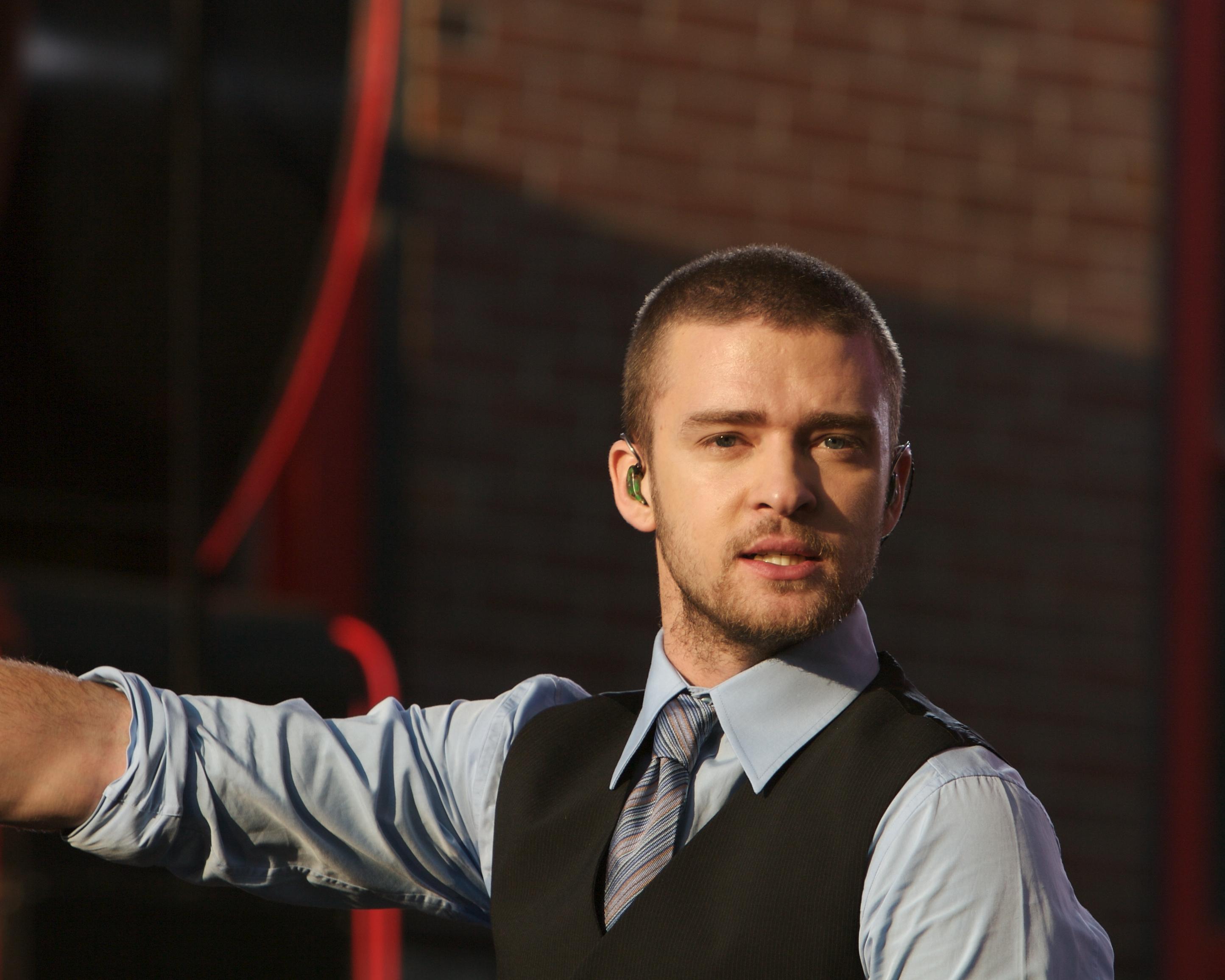This photographic image showcases a young white man with light brown, short hair and a high forehead. He sports a mustache and a bit of a beard, along with sandy-colored eyebrows and light blue eyes. His attire consists of a grey vest over a light blue collared shirt, with the sleeves rolled up to his elbows, revealing his bare arms. He dons a red and blue striped tie. A black earphone is visible in his left ear, and he gazes directly at the camera with his mouth slightly open, displaying mostly his bottom teeth. The lighting creates a shadow effect on one side of his face, giving it a dramatic look. In the background, a brown wall with two red stripes curves, and there's an impression of reddish, rectangular, and square shapes, possibly indicating an indoor setting. Some elements, like a window with a brown border, are subtly discernible but out of focus, adding to the depth of the scene.